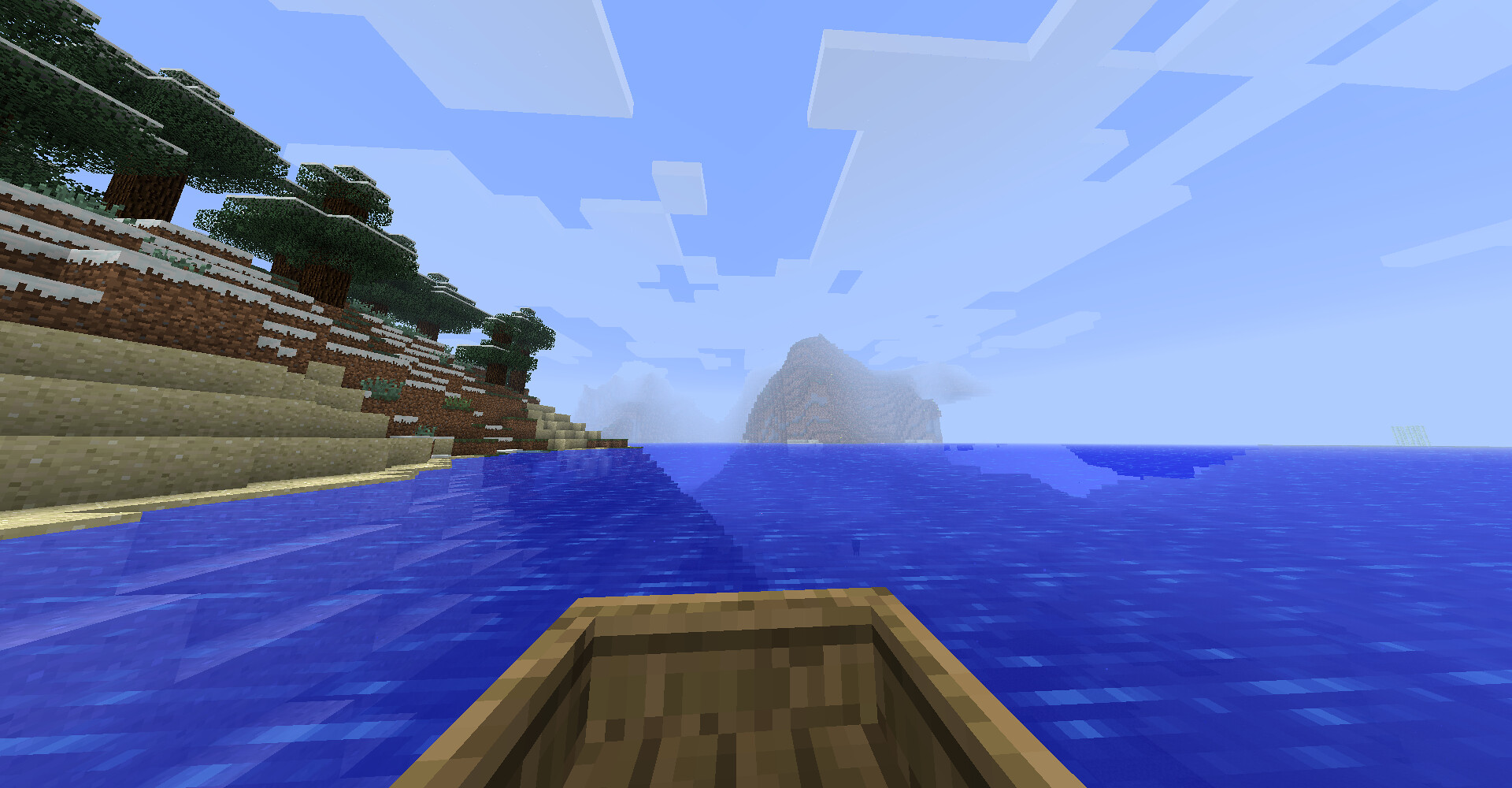This is a computer-generated image taken from within a popular video game, most likely Minecraft, given the distinct blocky, pixelated aesthetic reminiscent of both Roblox and Lego. The perspective places us in a small wooden rowboat, drifting in a vibrant blue ocean. In front, there's a towering gray mountain rising from the water like an island. On the left side of the scene, a terraced shoreline with layers of sand, dirt, and possibly some snow ascends to reveal stylized blocky trees. Above, a light blue sky dotted with stylized, translucent clouds frames this picturesque and nostalgic digital landscape.